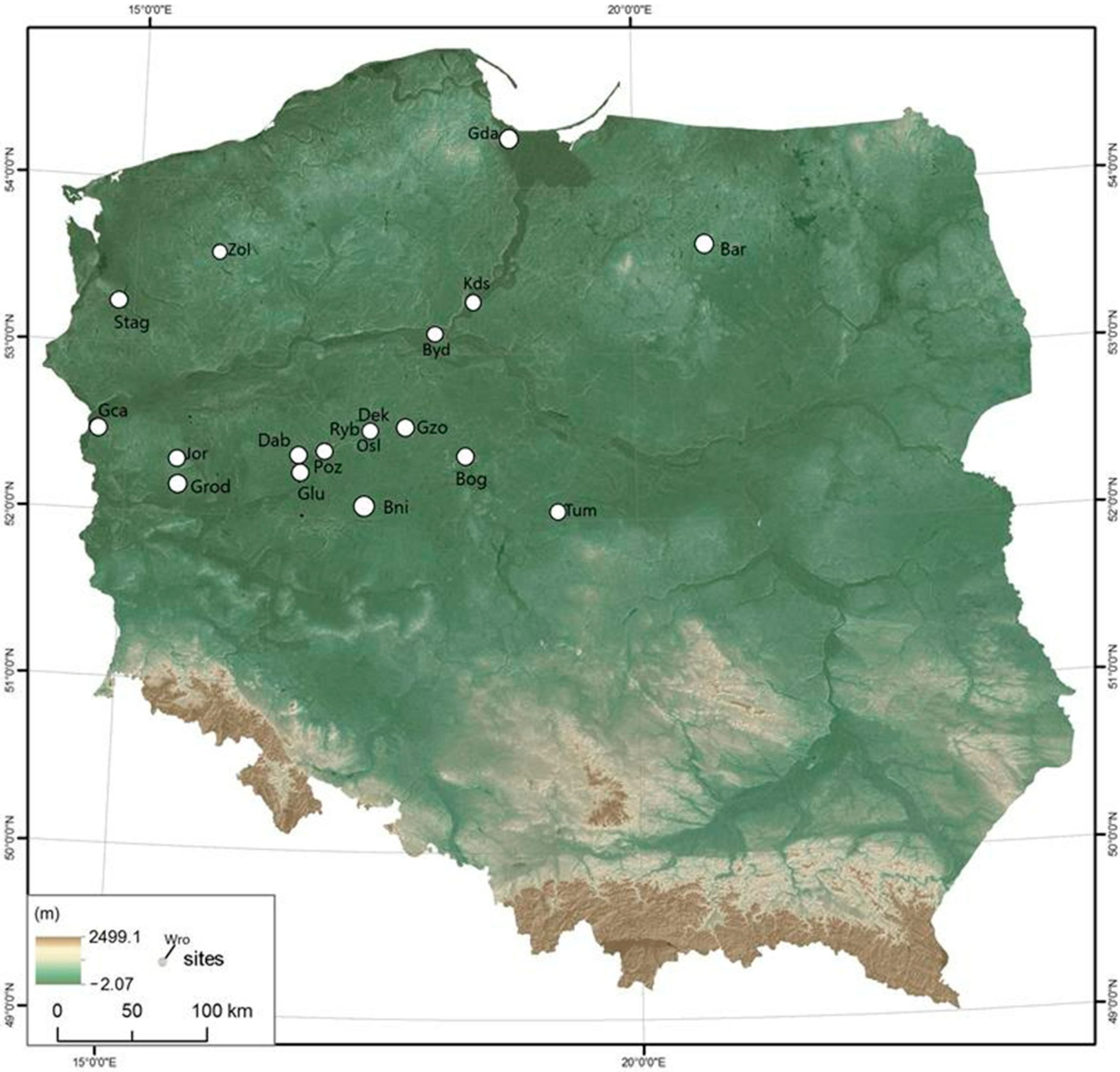This image is a detailed terrain map of an unidentified country, likely in Eastern Europe based on the features shown. The map uses various colors to indicate elevation, with green representing low-lying areas primarily in the northern part, transitioning to lighter and darker browns in the southern regions near the border, denoting higher elevations. The high elevations in the south seem to form a natural border. Key geographic elements include several rivers and white circles marking locations with three-letter abbreviations, possibly names of cities such as "Grodd," "Stagg," "Bahr," "Bog," "Zoll," "GCA," "GDA," "KDS," and "BYD." The map is square-shaped and includes a legend on the bottom left. It is bordered in black with latitude and longitude markings, providing coordinate references for navigation. Valleys are indicated by indentations along the rivers, primarily on the outskirts of the map.